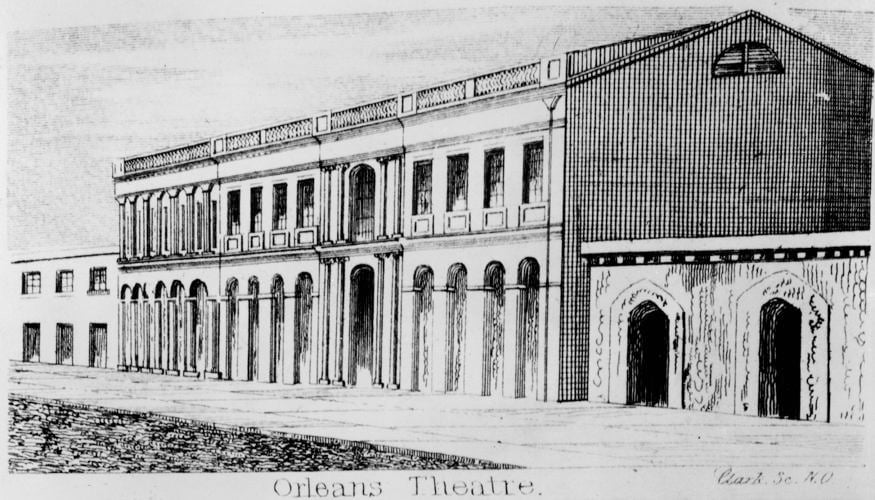This black-and-white drawing depicts the Orleans Theater, likely from the late 1800s to early 1900s. The central structure of the two-story building is prominent, flanked by two smaller sections. The main facade features multiple long archways on the first floor, with a significant primary archway entrance supported by four columns. The second floor showcases an array of windows, including a larger central window surrounded by thinner ones. The sketch indicates clear skies and a bright morning, with subtle shadows on the top right, suggesting sunlight. The foreground includes a wide walkway and a grassy field. Small buildings border the theater on both sides. There is an inscription at the bottom left that reads "Orleans Theater," and a partially legible name on the bottom right, possibly "Clark, S-E-N-O."